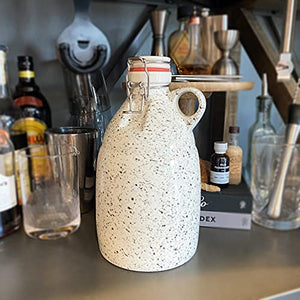This photograph captures a bar countertop adorned with various bartending essentials. Dominating the center is a vintage ceramic jug, speckled with black and gray, featuring a latching metal top and a circular, cut-out handle. The jug is accented with a red ring around its top. To its left sits a clear glass containing either water or another transparent liquid. Positioned behind these items are a bottle of Baileys and a black and yellow bottle, possibly Kahlua. Additionally, there are metal martini shakers, a muddler placed upside down in another glass, and various measuring tools, including slender shot measurers and an hourglass-shaped jigger, scattered around, hinting at the bartender's craft. The countertop itself has a grayish-brown hue, adding a rustic charm to the setting.